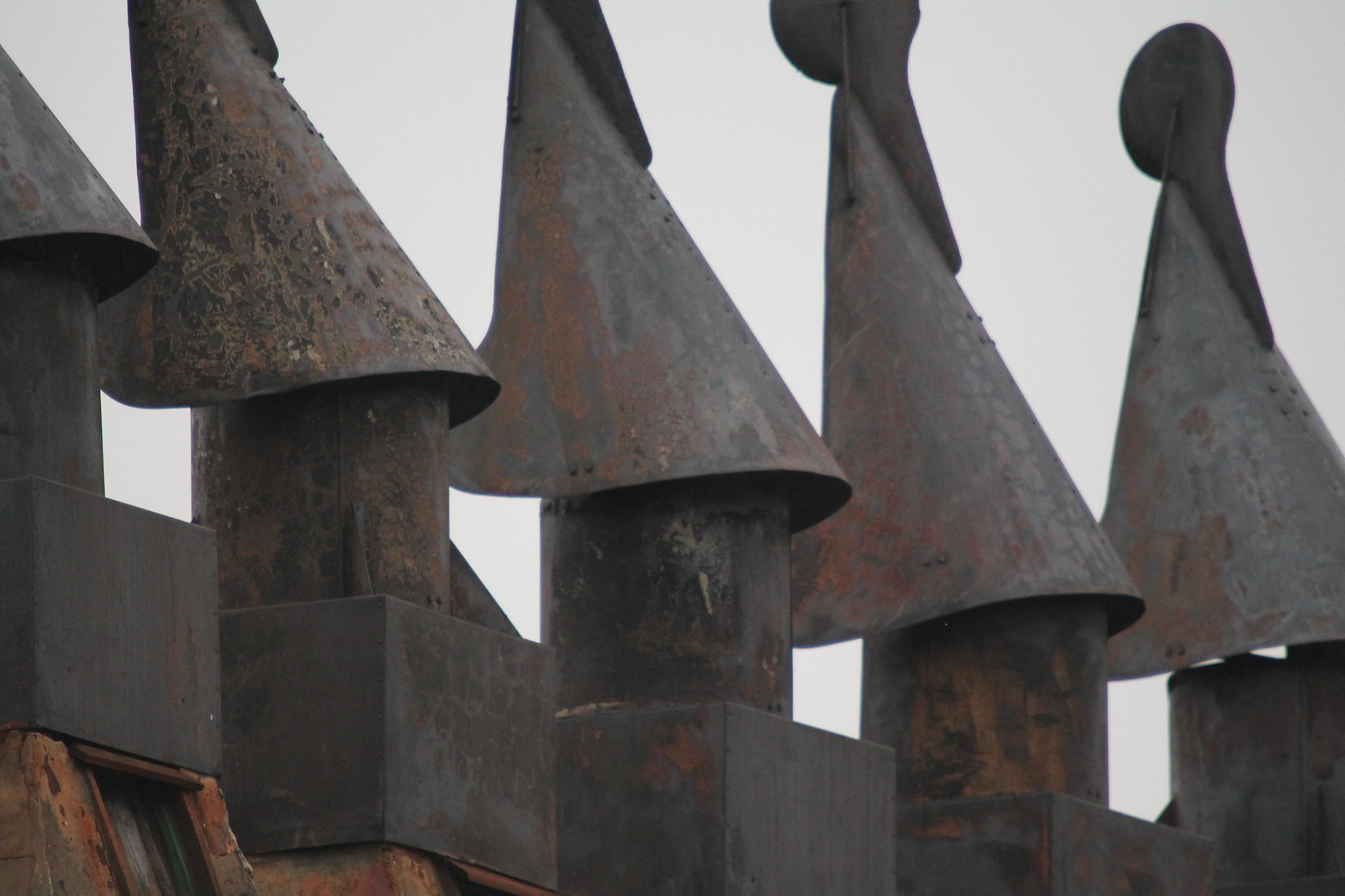This image depicts a close-up view of several steel chimneys on top of a roof, resembling an industrial setting. Each chimney consists of a square black metal base, transitioning into a cylindrical pipe. At the apex of each chimney is a rusted, dunce-cap-shaped cover, indicative of wear and age, with some displaying a reddish-brown hue due to rust. The covers also feature a small round embellishment with an arrow pointing down. There are five of these chimneys visible in the image, all aligned against a cloudy sky backdrop. The bottom left corner of the photo showcases a sloped, rusty brown wall, adding to the overall weathered and industrial feel of the scene.